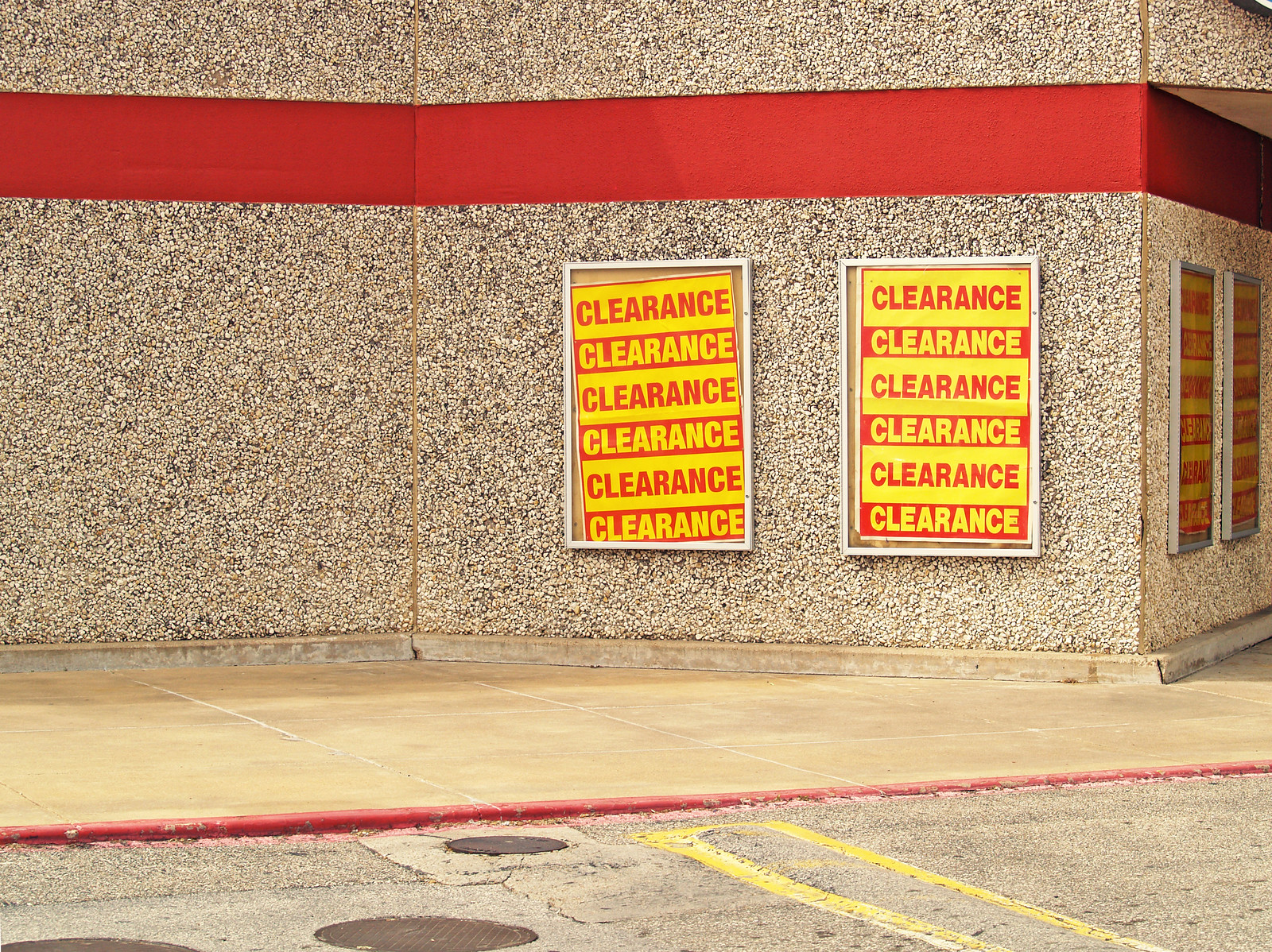This image captures the exterior of a building taken during daylight hours. The photograph, slightly zoomed in, focuses on the building's side façade. At the bottom, you can see a segment of the parking area featuring a red curb and adjacent sidewalk. The building’s wall appears to be constructed from small gravel-like material, giving it a textured appearance. A prominent red stripe runs horizontally across the top of the wall, adding a vivid color contrast. 

Two large rectangular signs are mounted on the right side of the wall. These signs feature alternating colors of red and yellow, with the word “CLEARANCE” repeatedly inscribed from top to bottom. The top section of each sign has a yellow background with red text, while the following section has a red background with yellow text, continuing in this pattern. This alternating design is mirrored on both signs. Another set of similar clearance signs can be seen around the building’s corner on the right, facing outward.